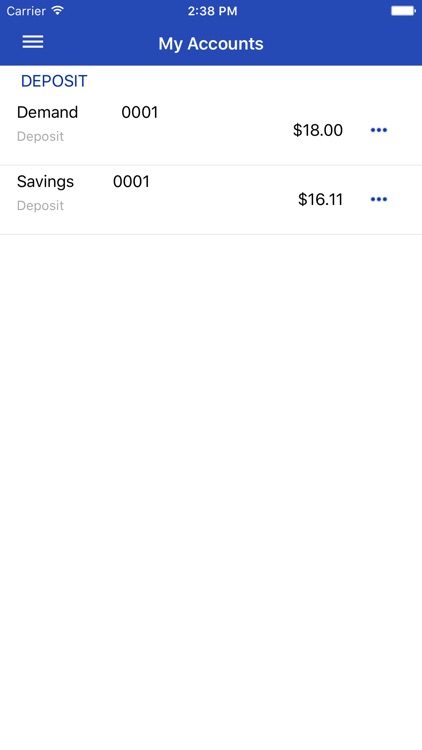A vertically-oriented screenshot of a banking app interface. The top section of the screen is a medium blue rectangle containing status symbols and navigation options. On the left side of this rectangle, the word "carrier" appears, indicative of placeholder text for a mobile network carrier. Next to it, icons for a Wi-Fi signal and the current time, 2:38 PM, are displayed. The right side shows a full battery symbol. 

Beneath this blue bar, a hamburger menu is positioned under the 'carrier' label, and centrally, the title "My Accounts" is prominently displayed. 

The body of the screenshot features two account listings. The first line reads "Deposit Demand 0001" in black text, with "Deposit" below it in gray. To the right of this, the account balance of $18.00 is shown, next to a three-dot menu icon indicating additional options. The second listing shows "Savings 0001" in black, with "Deposit" in gray underneath it. To its right, the balance is displayed as $16.11, also accompanied by a three-dot menu icon.

The remainder of the screen is white, extending down with no visible navigation bar or additional information, suggesting this is likely a placeholder or dummy data for a banking app. The specific bank or financial institution's branding and other identifying details are absent from this image.